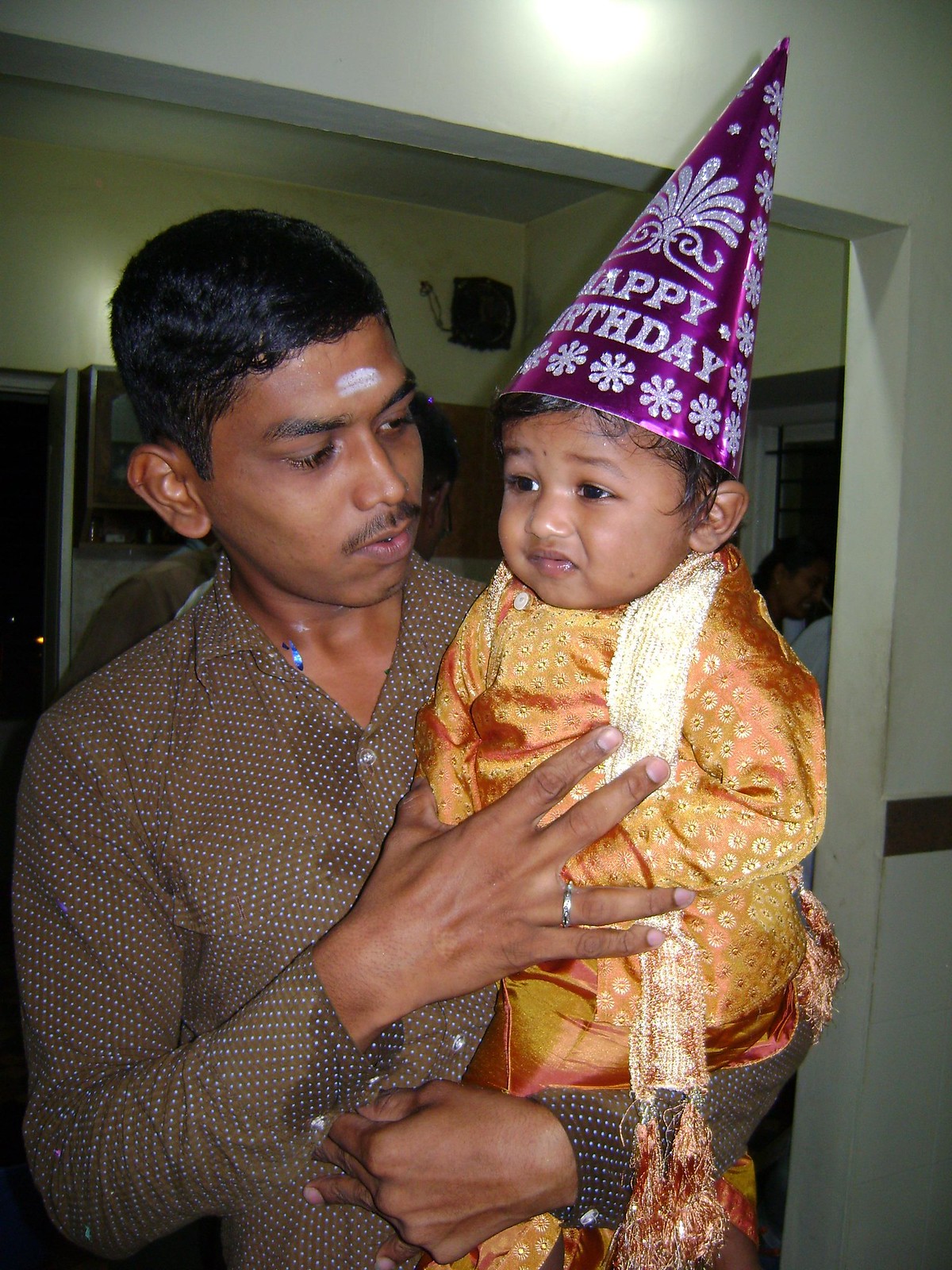The image depicts an Indian man, identifiable by the dark hair and a traditional white mark on his forehead, holding a baby. The man is dressed in a brown button-down collared shirt. The baby, who seems to be celebrating their first birthday, is wearing a bright orange outfit adorned with gold polka dots and a small gold shawl around the neck. The baby also wears a festive purple cone-shaped birthday hat decorated with silver flowers and glitter, with the words "Happy Birthday" inscribed in silver. Despite the festive attire, the baby appears somewhat unsettled and is looking away, seemingly disinterested or confused. The background suggests an indoor setting near a kitchen, with other individuals partially visible and possibly preparing for a meal, while the lighting indicates the use of a camera flash.